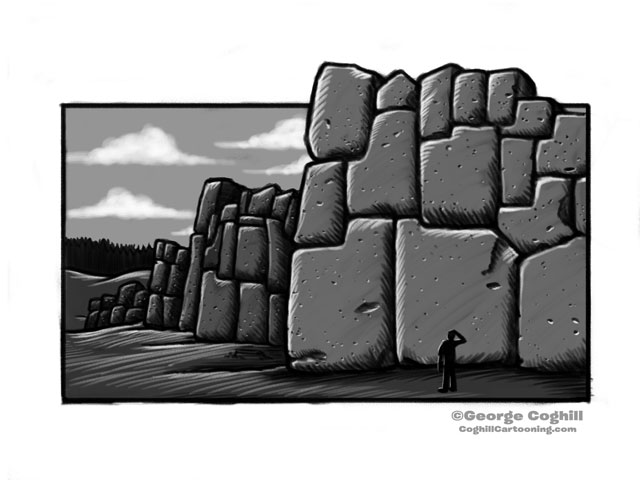This black-and-white cartoon drawing depicts a tiny man standing in the foreground, dwarfed by a colossal, towering wall of stacked stones that extends out of the top frame of the rectangular image. The stones, varied in shape and size, create a visually imposing structure, appearing meticulously arranged to form this massive wall. The ground below is depicted in shades of gray with white swirl lines, suggesting a dirt surface. The man, outlined in black, stands on the right side of the image, with his right arm bent and hand touching his head as if pondering or shading his eyes while looking up at the vast boulders. The background reveals a gray sky filled with white, puffy clouds and a forest of tall trees on a slope to the left. The entire scene is enclosed in a thick black border, enhancing its cartoonish aesthetic. At the bottom right corner of the image, the copyright mark and artist's name, "© George Coghill," along with the URL "coghillcartooning.com," are prominently displayed.